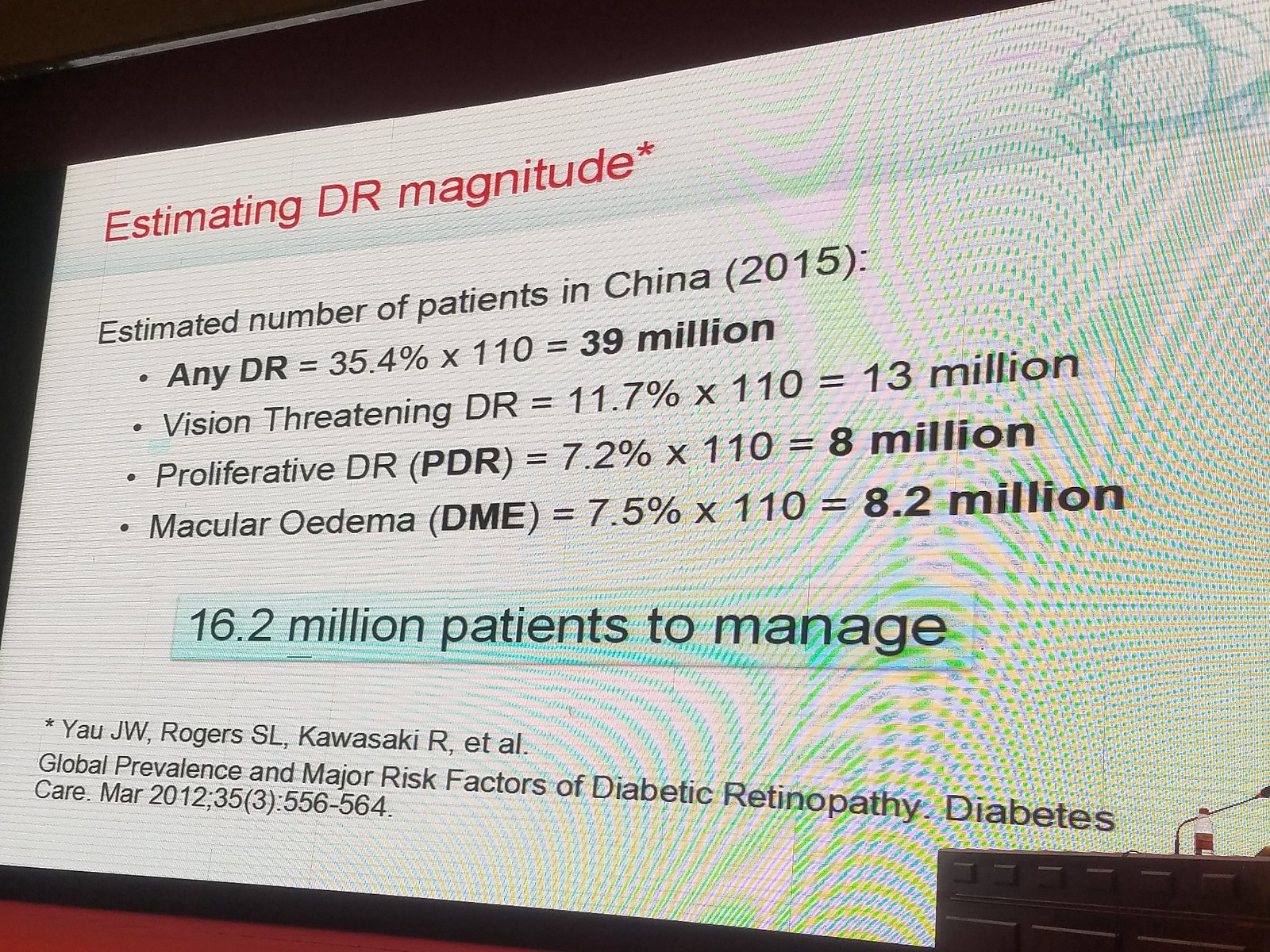The image is a large square photograph of a PowerPoint slide displayed on a white, drop-down projection screen at a medical meeting, possibly within a convention center. The photograph is taken from a slight angle below and to the right of the screen, revealing a black podium in the bottom right corner. A thin microphone and a water bottle are placed on the podium. The surrounding wall features black at the top and red at the bottom. 

The slide itself is primarily white, with a green and blue curvy pattern on the right side, possibly due to the angle of the photograph. At the top left of the slide, red text reads "Estimating DR Magnitude*". Below this, black text states "Estimated Number of Patients in China (2015)" with the following bullet points:
1. **Any DR** = 35.4% x 110 = **39 million**
2. Vision Threatening DR = 11.7% x 110 = 13 million
3. Proliferative **DR (PDR)** = 7.2% x 110 = **8 million**
4. Macular **Oedema (DME)** = 7.5% x 110 = **8.2 million**

A rectangular section with larger black text at the bottom of the slide declares "16.2 million patients to manage." At the very bottom, the source information is cited, corresponding to the asterisk in the title: "Yaw, J.W., Rogers, S.L., Kawasaki, R, et al. Global Prevalence and Major Risk Factors of Diabetic Retinopathy, Diabetes Care, March 2012, pp. 556-564."

The detailed caption thus provides a comprehensive description of the visual elements and the content of the slide, highlighting the key statistical information regarding diabetic retinopathy (DR) in China for the year 2015.